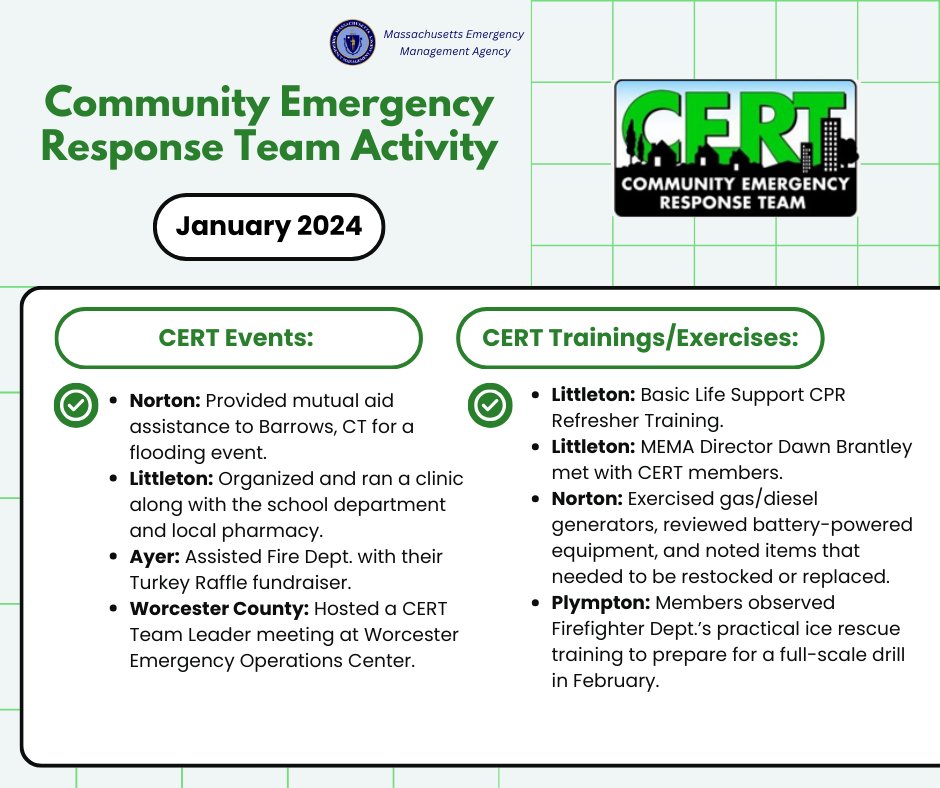The image is a detailed infoposter, likely derived from a computer interface, presenting information about an event organized by the Massachusetts Emergency Management Agency. At the top, the poster displays the agency's name along with the blue logo situated on the left. The main title, "Community Emergency Response Team Activity," appears prominently with the month and year "January 2024" indicated below. The acronym C.E.R.T. is mentioned, with its full form, Community Emergency Response Team, emphasized in green text.

The poster is divided into sections highlighting various activities and locations. "CERT Events" listed include Norton, Littleton, Ayer, and Worcester County, providing specific information for each location. For Norton, it includes events regarding exercise with gas and diesel generators and reviewing battery-powered equipment. Littleton is mentioned repeatedly, including basic life support CPR training. Additionally, Plimpton's activities involve members observing practical ice rescue training carried out by the fire department. The right section of the poster succinctly organizes "CERT Training and Exercises," again noting Littleton, Norton, and Plimpton. Another noteworthy point is a mention of mutual aid provided to Barrows, Connecticut, for a flooding event.

In summary, the image is an informative and organized breakdown of the Community Emergency Response Team activities and training sessions scheduled for January 2024 across several Massachusetts locations, emphasizing the detailed preparedness and training support provided by the organization.